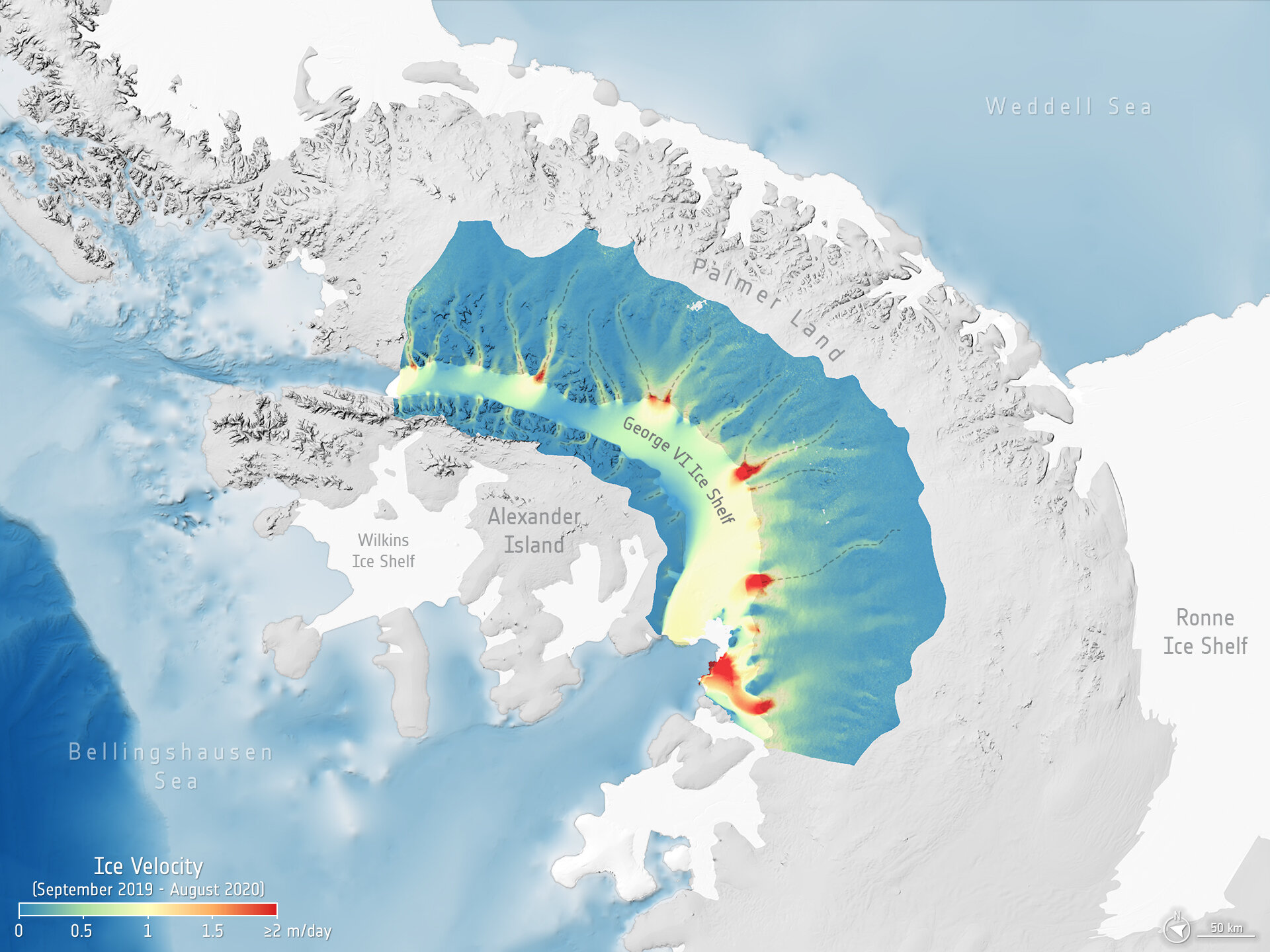This image is a detailed map depicting ice velocity from September 2019 through August 2020. Dominated by shades of light blue, white, and very light gray, it includes various notable regions marked on it. These regions include Wilkins Ice Shelf and Alexander Island prominently in the center, with the George VI Ice Shelf also highlighted, featuring pockets of yellow, green, and red indicating higher velocities. The top right of the map labels the Weddell Sea, while the bottom right notes the Ronne Ice Shelf. The bottom left corner identifies the Bellinghausen Sea, and nearby is Palmer Land. The map includes a velocity scale that transitions from dark blue (indicating 0) to red (indicating velocities greater than or equal to 2 meters per day). Additionally, a graph in the lower left corner displays this scale in colors from blue to red, with intermediate bands of yellow, orange, and green, corresponding to varying ice velocities across the mapped regions. The bottom right corner features a compass for distance, marked at 50 kilometers.